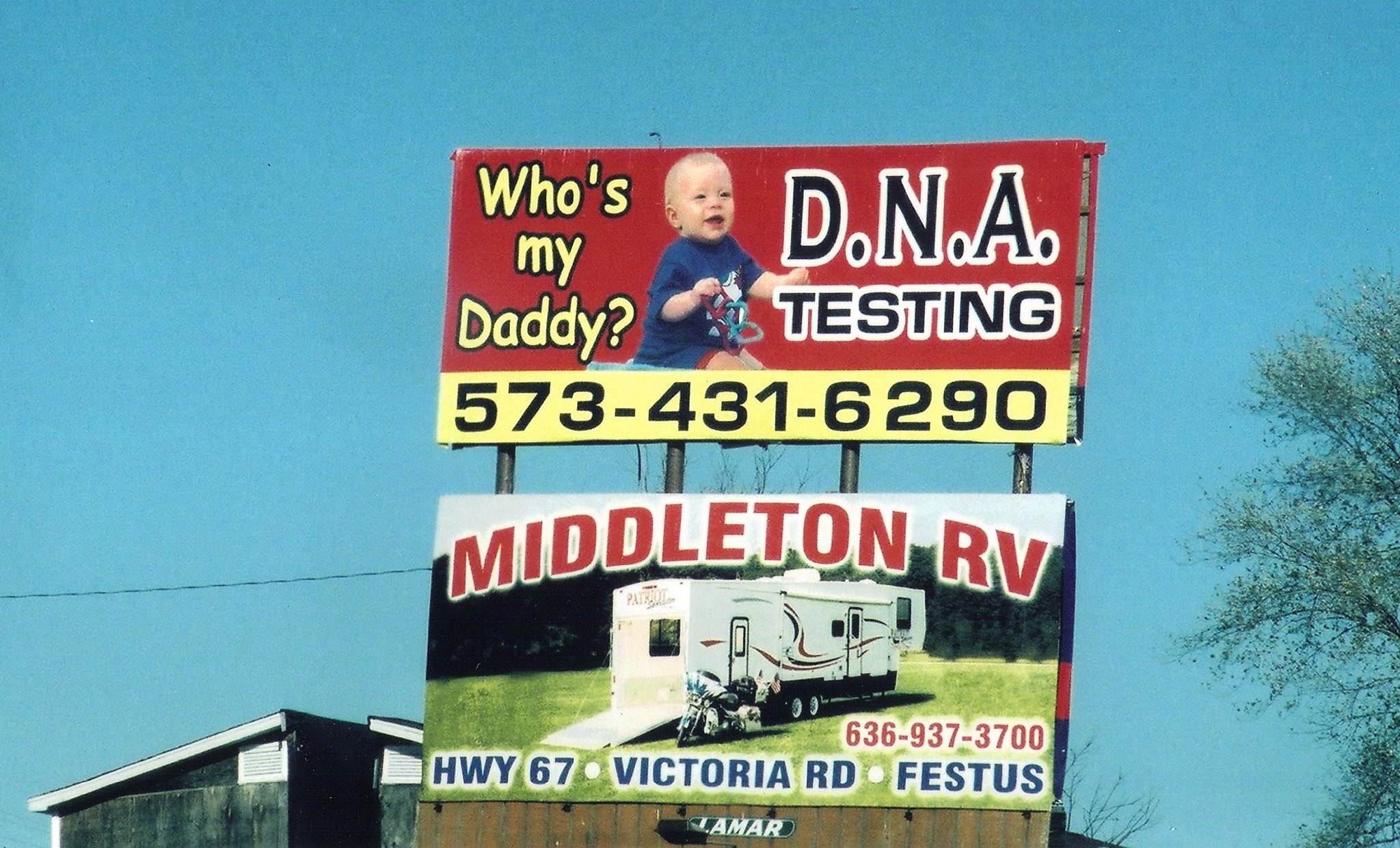In the photograph, a vibrant, crystal-clear blue sky devoid of clouds forms the backdrop. Dominating the center of the image is a double-stacked billboard supported by four metal pipes. The top billboard, which is predominantly red with a yellow bottom third, features a picture of a baby in a blue shirt. On the left side, the text reads "Who's My Daddy?" in yellow font, while on the right, in black font, it states "DNA Testing" along with the phone number "573-431-6290" across the bottom. Below this, another rectangular billboard advertises Middleton RV, showcasing a white RV trailer parked on lush green grass. The words "Middleton RV" appear in bold red font at the top, and at the bottom, in smaller black font, it lists "Highway 67, Victoria Road, Festus" with the phone number "636-937-3700" above it in red. In the lower left corner of the photo, a house with an A-frame roof is partially visible, and the far right edge is marked by the presence of several trees.